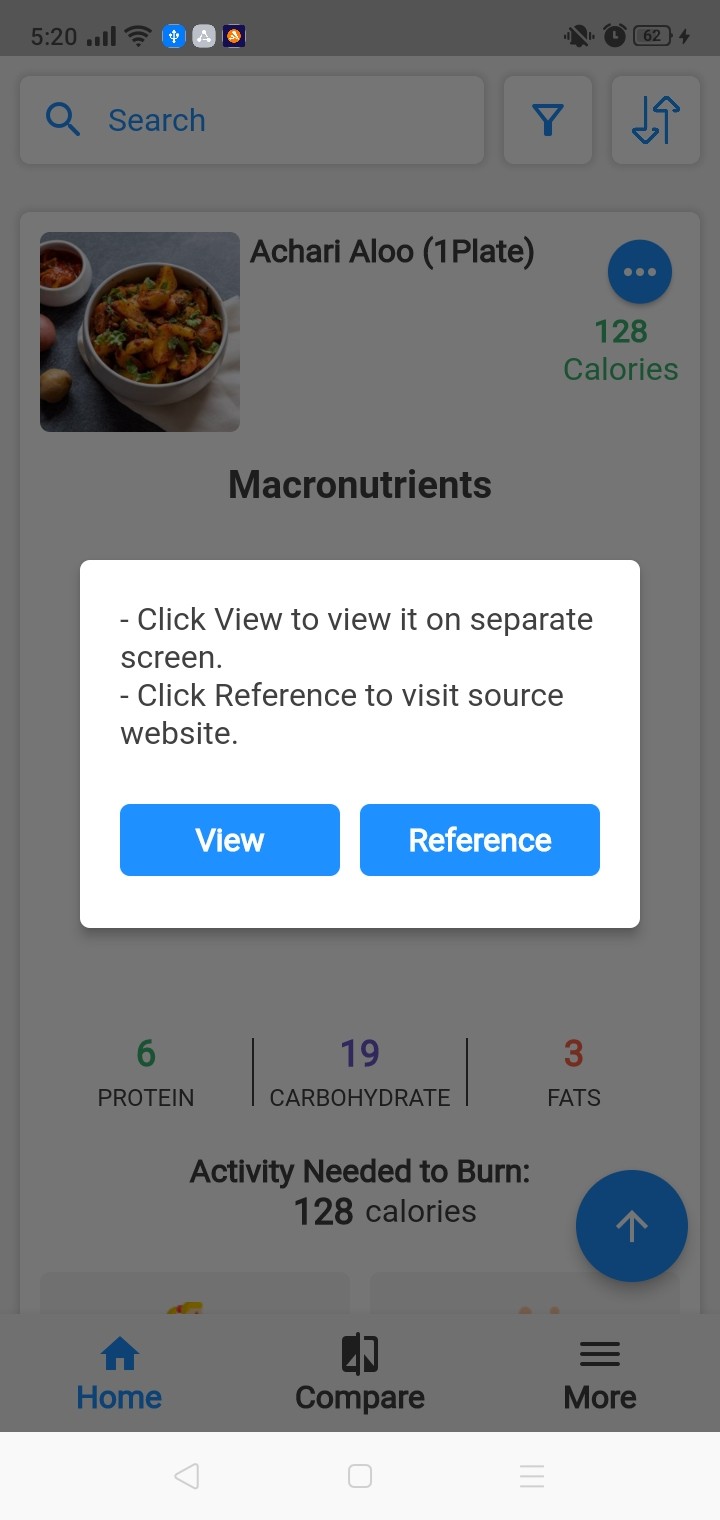This is a detailed screen capture of a smartphone displaying various pieces of information. The time shown on the phone is 5:20, with full signal bars and the battery level at 62%. There are multiple notifications indicated at the top of the screen which the user has not yet checked. 

The main content of the screen is about a dish called "Curry Aloo," which is accompanied by a small image of the completed dish. The nutritional information for one plate of Curry Aloo is detailed as follows: it has 128 calories, with a macronutrient breakdown of 6 grams of protein, 19 grams of carbohydrates, and 3 grams of fats. Additionally, it mentions the activity required to burn these 128 calories, although further details are cut off in this capture.

There is also a white pop-up window at the bottom of the screen with options for the user to either "Click View" to view the information on a separate screen or "Click Reference" to visit the source website, awaiting the user's choice.